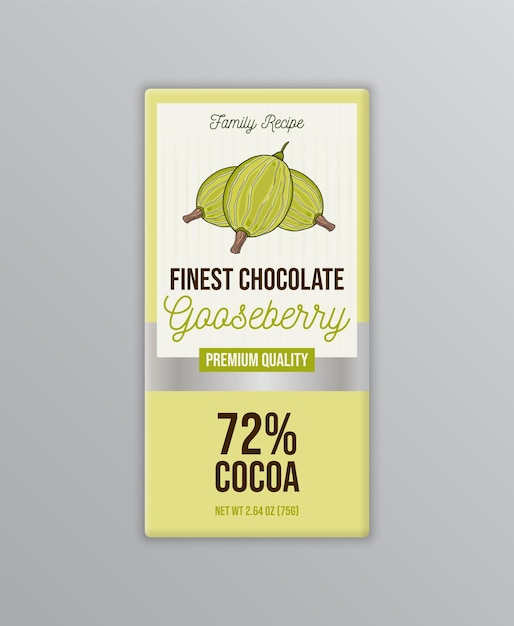The image depicts a computer-rendered chocolate bar package set against a light gray background. The packaging is vertically oriented and two and a half times as tall as it is wide, with a predominantly light yellowish-green, muted, pastelish color scheme. The top portion features a large, portrait-oriented white rectangle covering the top 60% of the wrapper. At the top of this white rectangle is a small italicized brown text reading "Family Recipe."

Below this, there are three overlapping gooseberries illustrated in darker yellowish-green, resembling small melons with brown stems. Following the gooseberries, the text "Finest Chocolate" is printed in all caps in dark brown, and underneath it, the word "Gooseberry" is written in cursive in a dark yellow color.

A silver shiny strip runs horizontally across the lower middle section of the packaging. Below this strip, there is a smaller darker yellow-green rectangle containing the text "Premium Quality" in white. Finally, the bottom portion of the package features bold, large dark brown text stating "72% cacao," and below that, "NET WT 2.64 OZ (75g)" in the same dark yellow color used for "Gooseberry."